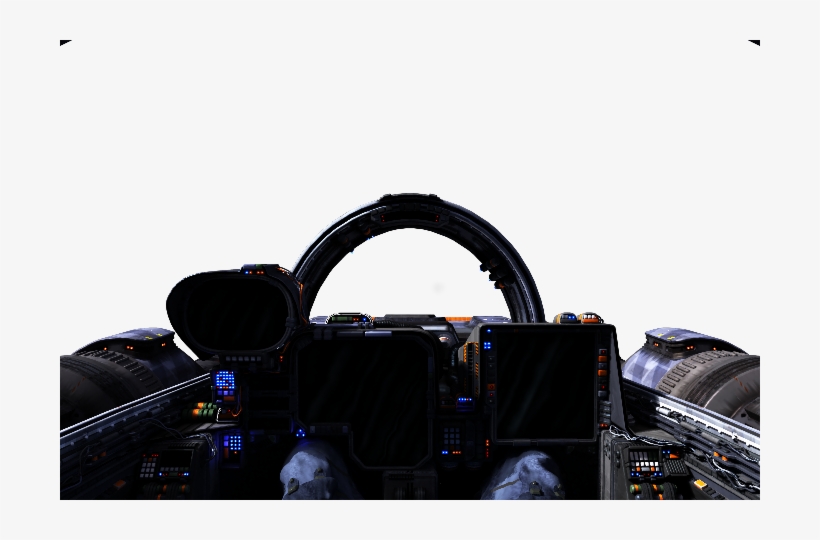The image depicts the interior of a compact cockpit against a stark, completely white background, framed by small black triangles at the upper left and right corners. Centrally positioned at the bottom of the image is a metal terminal, indicative of various control mechanisms. The console is adorned with an array of buttons in red, white, and blue; some of these are lit, while others remain dark. The console features three monitors: a circular screen on the left, a larger central screen, and a smaller square one on the right. Each screen is surrounded by the aforementioned multicolored buttons, contributing to the high-tech, possibly futuristic, or science fiction vibe of the setup. The presence of a half-circle structure at the front of the console further suggests this might be the control panel of either a submarine or an aerial vehicle. Despite its advanced appearance, the specific functions of the controls and screens remain indistinguishable.